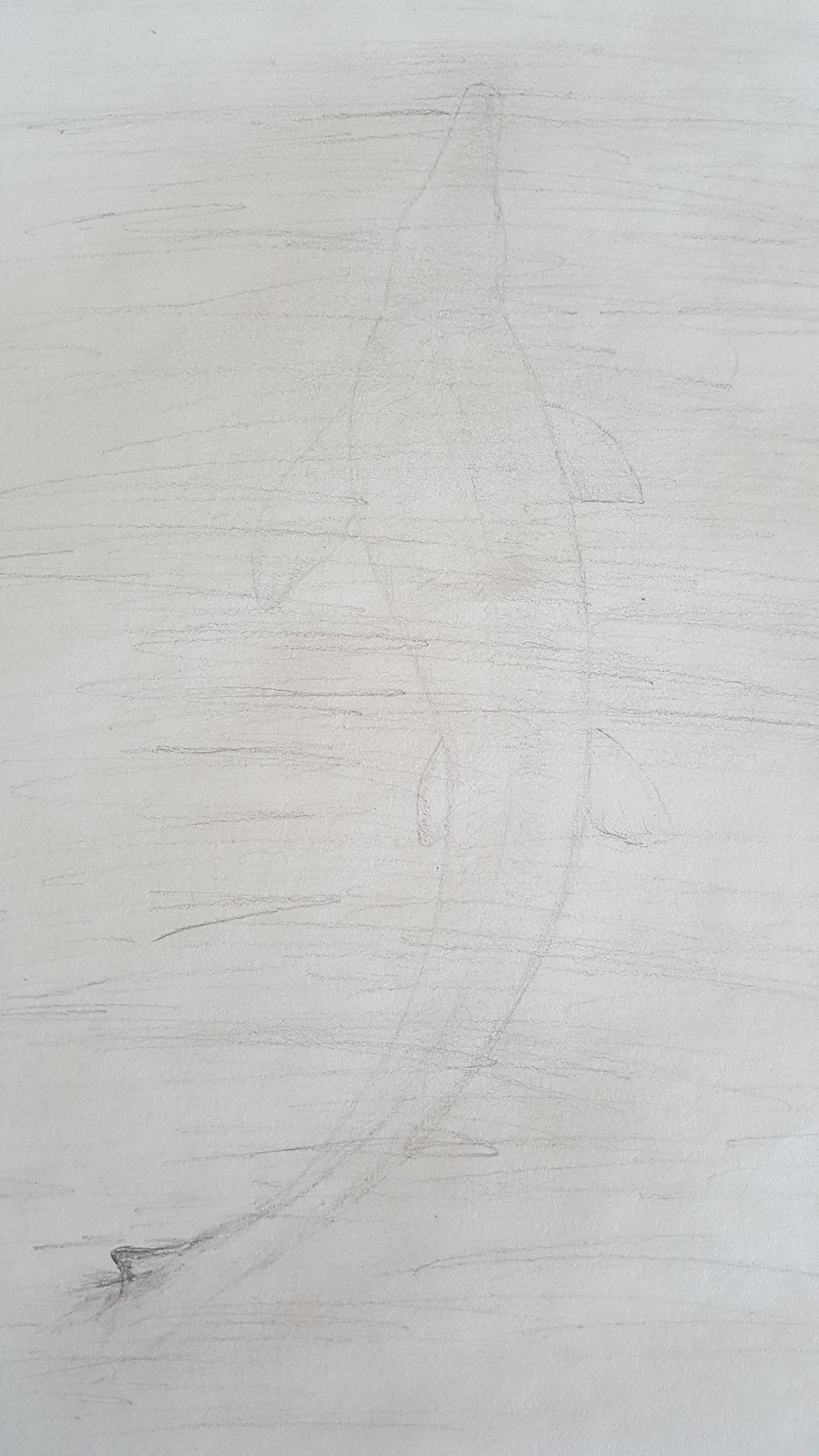A light gray piece of paper serves as the canvas for a pencil drawing. The most prominent feature is a faint, abstract shape resembling an alligator. This shape can be deciphered by its long nose extending into a body, with small feet adorning each side and a lengthy tail trailing behind. The tail is heavily emphasized in dark black, with the artist repeatedly sketching over this section to create a stark contrast to the lighter, more subtle pencil markings that make up the rest of the figure. Along the sides of the paper, sporadic scribbles add a sense of spontaneity and unfinished detail to the overall composition.